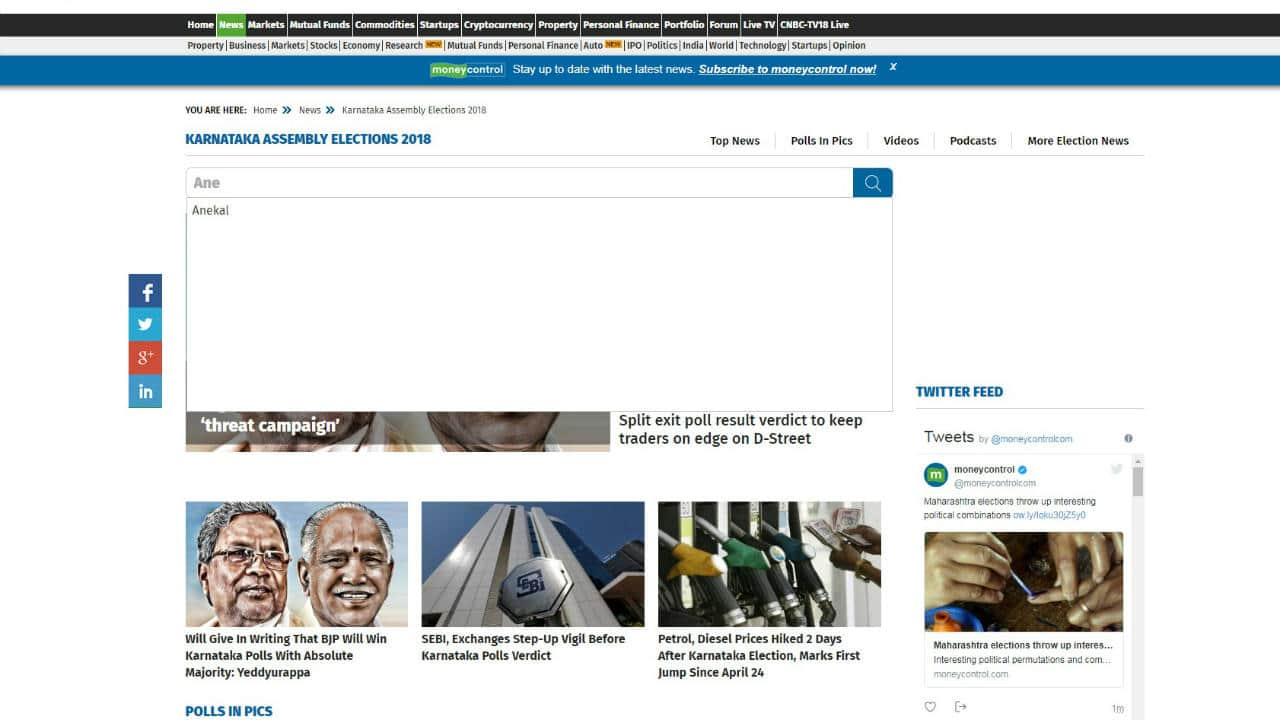This image is a detailed screenshot of a web page, showcasing multiple layers and design elements. At the very top, the border is black, followed by a gray section, and then a blue section beneath it. The text is small, making it difficult to identify the website clearly. However, the navigation bar on the black background includes links such as "Home," "News," "Strategies," "Property," and "Personal Finance." 

A secondary header suggests "Money Central" might be the website's name, as it prominently states, "Sign up to date with the latest news" and "Subscribe to Money Central now" in white text.

The main content area of the page has a white background and appears to be a news site. At the top, in blue, it reads, "Karnataka Assembly Elections 2018," followed by a search box and a dropdown menu that obscures part of the content. Visible at the bottom row of stories are three photos. One photo prominently features gas pumps with the caption, "Petrol diesel prices hiked two days after Karnataka election marks first jump since April 24th." This strongly suggests that recent elections and fuel price hikes are significant topics featured on the site.